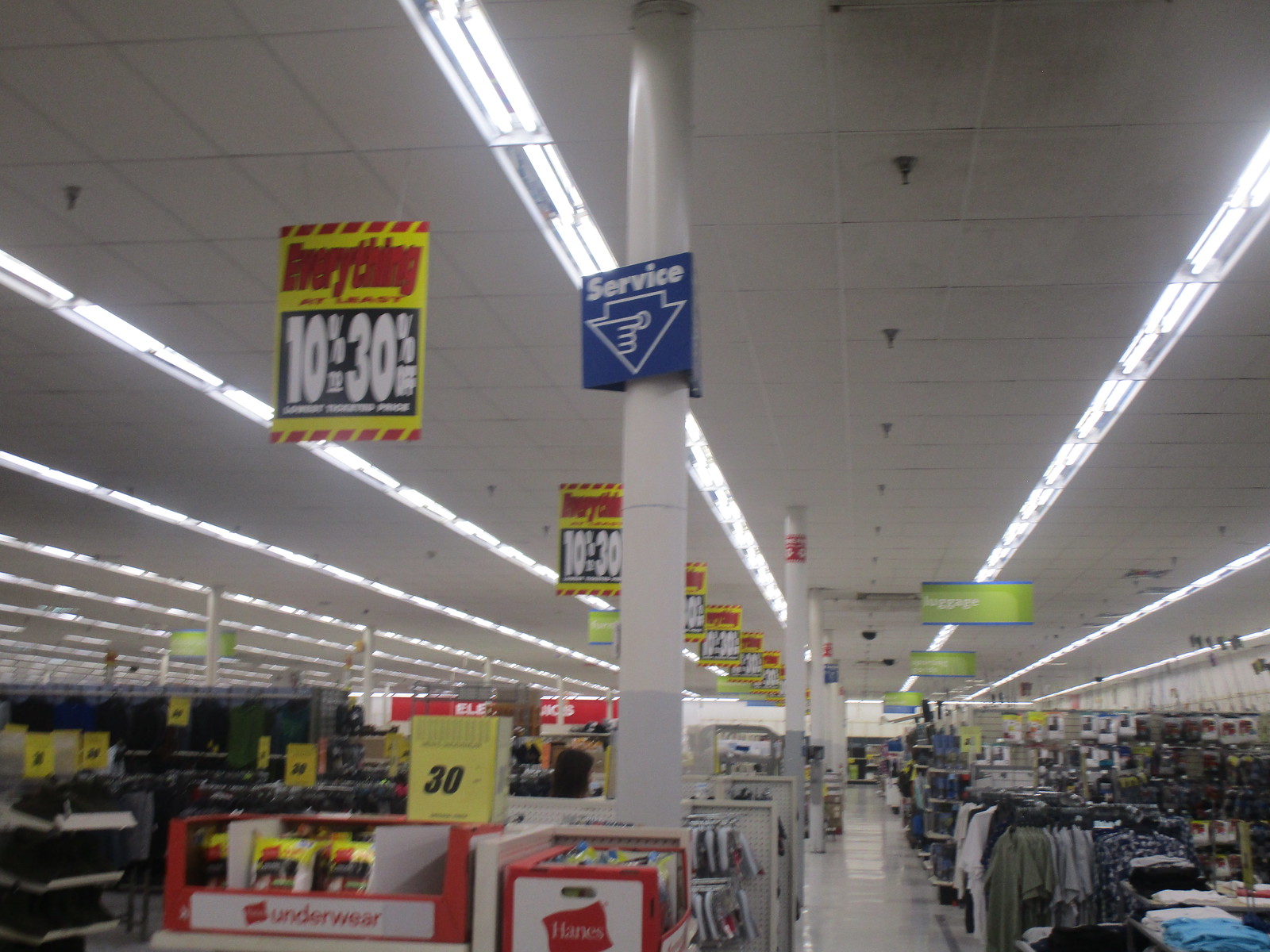This photo captures the bustling aisle of a large department store, likely a big-box chain. The viewpoint is from a standing position, looking directly down a well-lit aisle. On the left side of the aisle, there's a section dedicated to clothing, prominently featuring packages of Hanes underwear. To the right, an array of apparel items such as shirts and pants are neatly displayed. In the distance, a display of socks is visible, adding to the comprehensive selection of garments.

The ceiling is adorned with clean, white ceiling tiles, contributing to the store's bright and organized ambiance. Several square signs hang down from the ceiling, featuring a vivid color scheme of yellow, black, red, and white. These signs announce discounts ranging from 10% to 30% off, enhancing the shopper's visual experience with enticing deals.

Additionally, a blue sign attached to a nearby pole reads "Service" and depicts a hand pressing a button. This suggests the presence of a service request button at the pole's base, offering customers the convenience of summoning assistance when needed. The overall scene is indicative of a typical department store environment, structured to facilitate an efficient and enjoyable shopping experience.